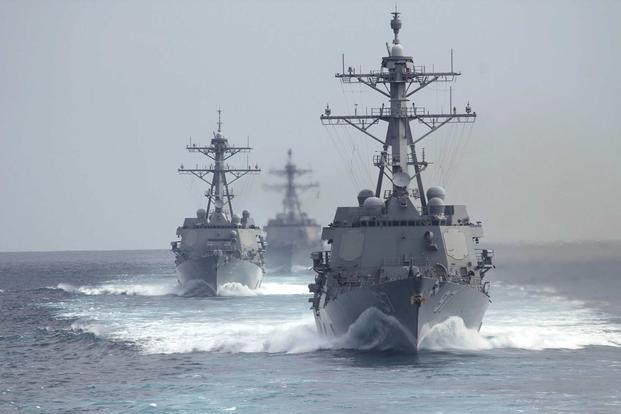This horizontally aligned rectangular image captures a silvery, gray-toned seascape featuring three large military ships, which resemble oil freighters. The upper part of the picture is dominated by a solid, medium gray, blue-tinted sky, while the lower part shows a similarly colored ocean with streaks of white waves created by the moving ships.

Centered slightly off to the right and closest to the camera, the foremost ship is depicted in sharp focus, generating visible white waves as it advances. This ship, like its companions, is entirely gray and appears devoid of any personnel on deck. It’s equipped with a metal mast supporting various antennas and four radar dome structures on top.

Behind the lead vessel, another ship is clearly visible but set back, followed by a third, slightly to the right and more distant, appearing blurry and less distinct. All three ships are identical in design, suggesting a fleet, and are uniformly gray. As they speed forward through the gray and silvery waters, their progress is marked by the tumultuous waves in their wake, capturing the dynamic energy of their motion in this striking, monochromatic daytime scene.